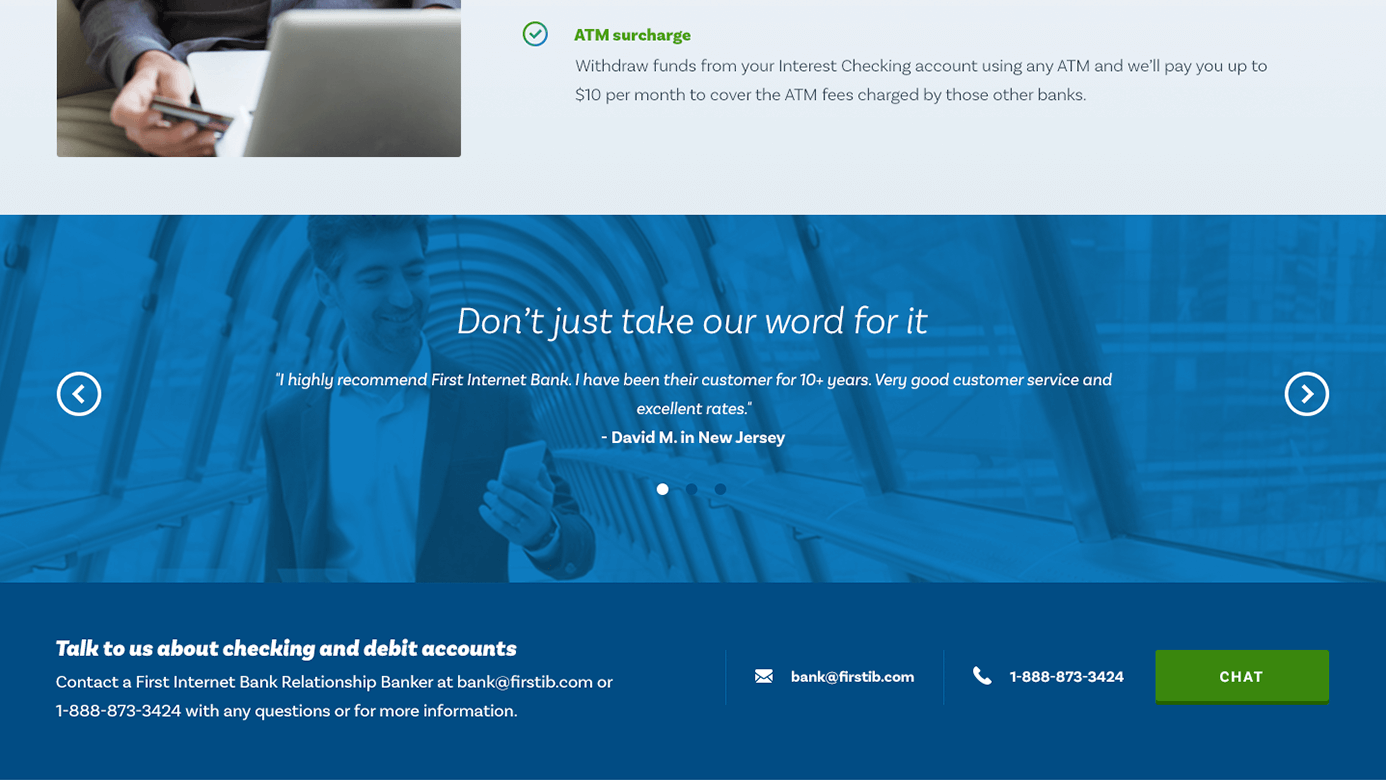This image is a detailed screenshot of a bank services page, featuring various sections and interactive elements. 

At the top of the image lies a gray horizontal bar. In the upper-left corner, there is a small thumbnail picture depicting an individual holding a phone and a laptop. Adjacent to this thumbnail is the prominent heading "ATM Surcharge," which is accentuated by blue and green checkboxes. Directly below this heading is a succinct message: "Withdraw funds from your interest checking account using any ATM and we'll reimburse you up to $10 per month to cover the ATM fees charged by those other banks."

Beneath the gray bar is a larger blue section with a background image of a person walking through a tunnel walkway, engrossed in their phone. On either side of this background image, there are left and right arrows designed to toggle between different testimonial statements. The current testimonial displayed reads, "Don't just take our word for it." Following this heading, in smaller text, a satisfied customer named David M. from New Jersey shares his experience: "I highly recommend First Internet Bank. I have been their customer for 10 plus years. Very good customer service and excellent rates." There are a total of three quotes available for viewing in this section.

Further down, a darker blue bar appears with the heading, "Talk to us about checking and debt accounts," accompanied by smaller text providing additional details. To the right of this heading, at the bottom of the blue bar, there are contact options displayed. These include the bank’s email address and phone number. Additionally, there is a green rectangular button labeled "Chat," providing an option for live assistance.